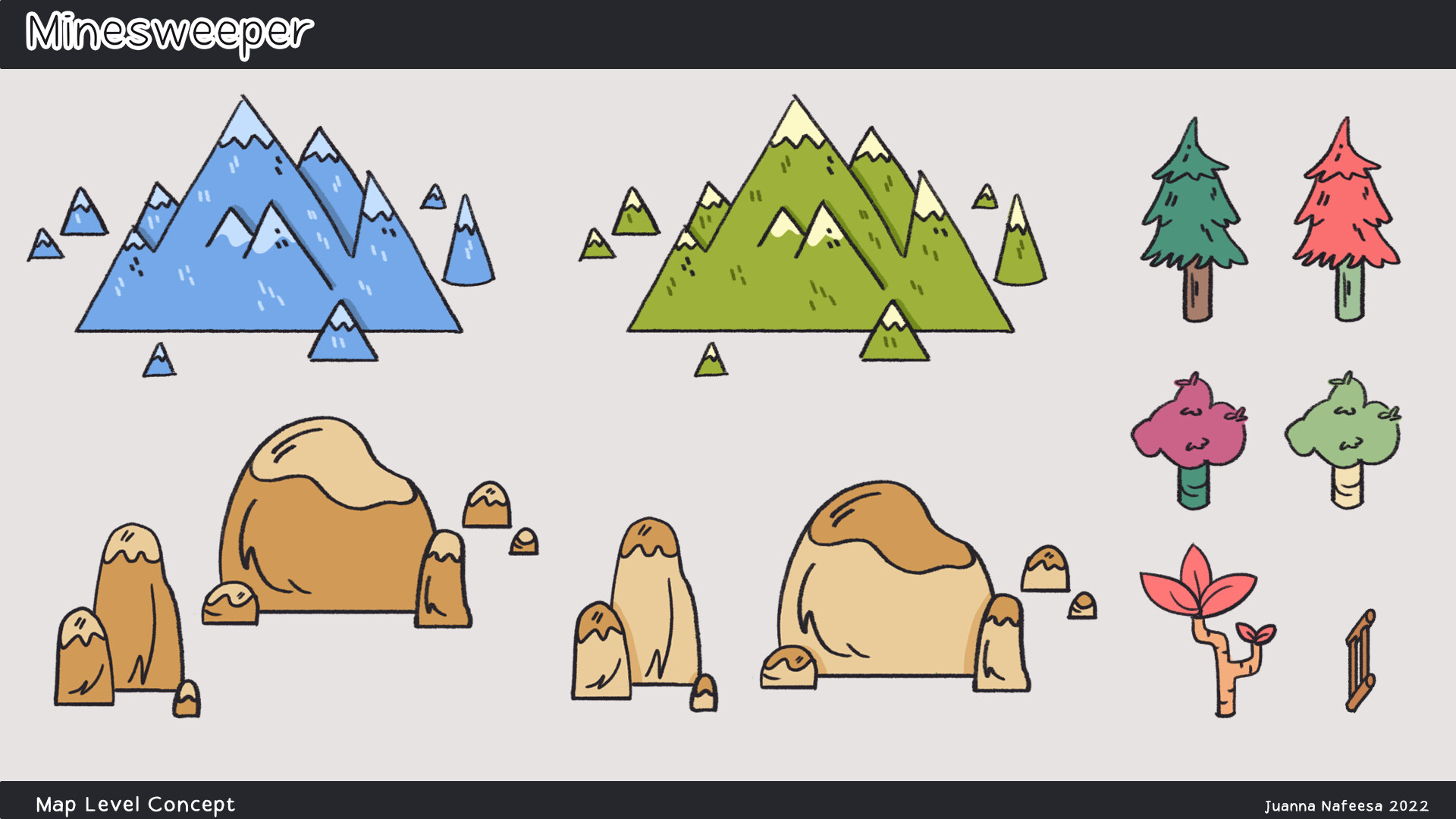This is a detailed illustration titled "Minesweeper" featuring a combination of vibrant and pastel hand-drawn elements. Across the top, a black strip includes the title "Minesweeper" in contrasting black and white lettering. The central part of the image showcases two crudely drawn mountain ranges—one blue with snowy ice caps, and another green with light creamy colored peaks. Below these mountains are two rock formations: one a darker brown and the other a lighter beige with brown accents.

To the right of the mountains, there are two pine trees; one green with a brown trunk and the other red with a green trunk. Directly beneath these pine trees, there's a pair of smaller, differently styled trees: one pink with a green trunk and another green with a tan trunk. Under these smaller trees, a small plant or branch with budding leaves is illustrated, colored red. Next to this plant, on the very right side, appears to be a small brown wooden fence-like structure.

At the bottom of the image, a black strip carries the text "Map Level Concept." In the bottom right-hand corner, the artist's name "Juana Nafisa 2022" is inscribed, marking the creation of this detailed and evocative illustration.